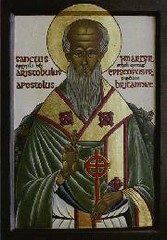The image is a small, rectangular, framed piece, about the size of a stamp, depicting an old icon from an Orthodox Church. It features a religious figure, possibly a character from biblical literature, drawn in an older, somewhat stylized manner. The man at the center has a long, gray beard, balding head with short gray hair on the sides, and brown skin. He is adorned with a gold halo that extends onto the thin black frame of the image. The figure wears a dark green robe with a gold sash that has red trim and a red cross on it. Additionally, he holds another red cross on a staff close to his chest with his left hand. His right hand is raised in a gesture, with two fingers up and the rest down, directed towards the viewer. There is text in a foreign language in red situated above his shoulders on the top left and top right corners of the image.